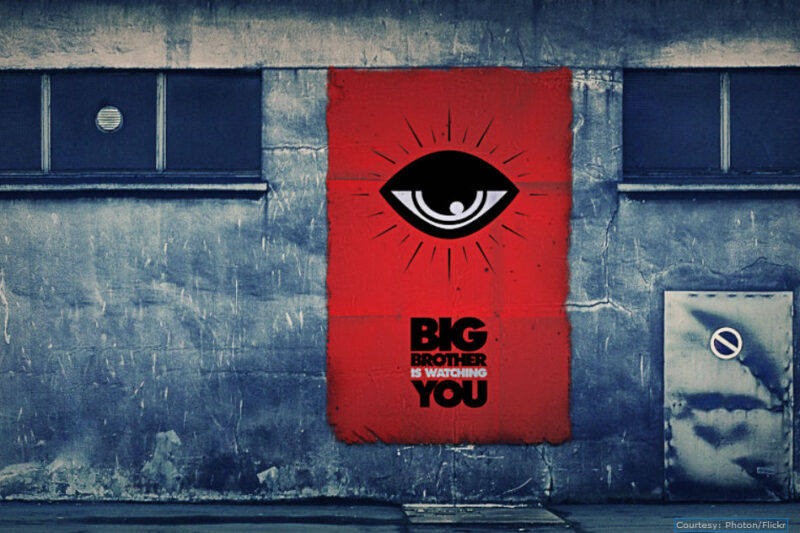This photographic image captures a stark and evocative outdoor setting. Dominating the scene is a prominent red sign affixed to the gray, white-marked wall of a building. The sign features a striking graphic of a black eye with arrows or rays radiating from its center, symbolizing vigilance. In bold black and white text, the sign declares, “Big Brother is watching you.” The sign is centrally positioned between two windows; the left window bears a white sticker, and both windows are adorned with multiple pings—three on the left and two on the right. Significantly, to the bottom right of the image, there is a poster displaying a photo of a mouth crossed by a "do not enter" symbol, a circle with a diagonal line. The scene is devoid of people, underscoring the unsettling, surveillant atmosphere.